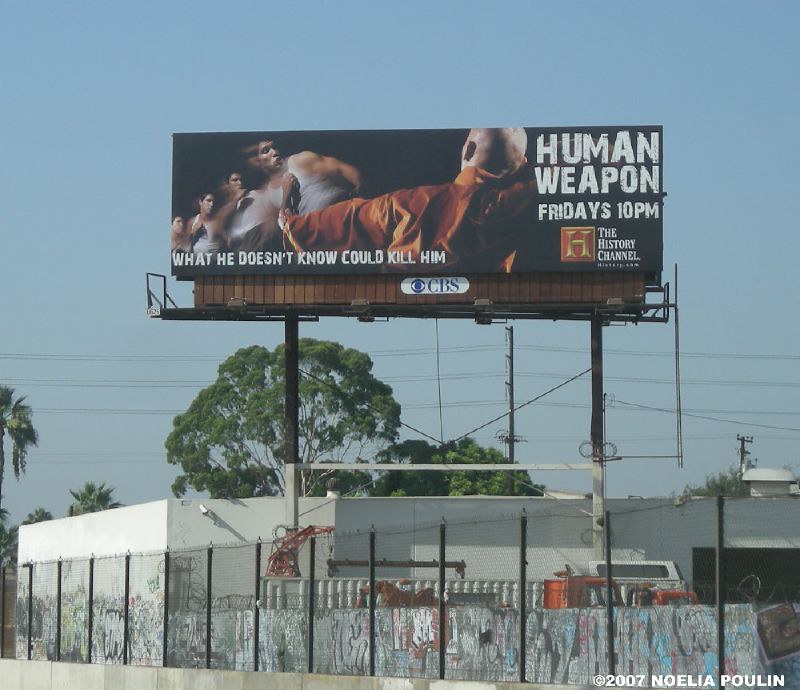The photograph captures an outdoor scene featuring a vivid medium blue sky devoid of clouds. Dominating the top portion is a prominent billboard. The right side of the billboard showcases the text "Human Weapon Fridays 10 p.m." besides an emblem of a gold 'H' on a red square background, signifying the History Channel. The billboard's tagline, "What he doesn't know could kill him," is also clearly visible.

In the visual narrative, the back of a bald man donning a rust-colored robe is prominently displayed. He appears to be in a dynamic pose, potentially kicking towards another man opposite him who is shirtless. Below this action scene, the acronym "CBS" is inscribed.

Beneath the billboard and grounding the image is a single-story building with white-painted brick, featuring some kind of paneling along its fence, which is likely where considerable graffiti is scrawled. The photograph is credited at the bottom with the text "© 2007 Noelia Poulin".